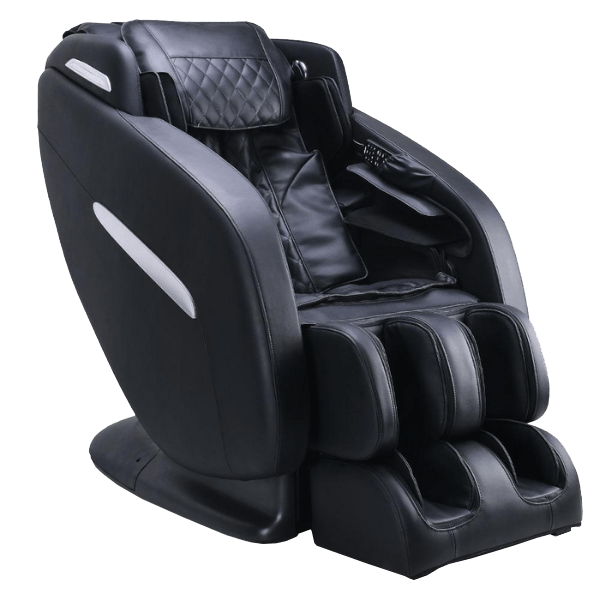The image depicts a modern-day, pod-shaped massage chair displayed against a pure white background. The chair, made entirely of sleek, patent black leather, features a luxurious design reminiscent of high-end merchandise seen in a Sharper Image catalog. Its contours are angular, resembling a tic-tac dispenser, and it encompasses a thick, sturdy base. The seat transitions seamlessly into a sloped backrest adorned with small massage nodules and a diamond-patterned head pad for optimal comfort. The chair also includes built-in footrests with two grooves designed to cradle the legs and feet, providing a comprehensive leg massage. On the right-hand side of the chair, there is a conveniently placed pocket for storing the remote control, ensuring ease of use. The armrests are integrated within the angled sides of the chair, adding to its streamlined, futuristic aesthetic.